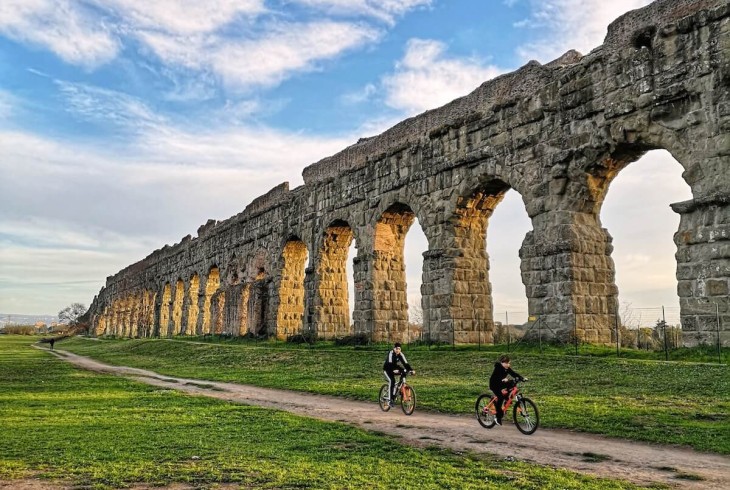This photograph captures an outdoor scene featuring two bicycle riders, presumably a woman in the front and a man behind her, riding towards the bottom right corner of the image on a dirt road. They are on orange bikes, and the road is flanked by cut grass fields that aren't particularly tall. To the riders' left (the photograph's right) stands an impressive and ancient stone structure, identified as the old Roman aqueduct in the Park of the Aqueducts. This aqueduct stretches far into the background, showcasing approximately 15 to 20 arches, each formed from large stone bricks, some of which appear weathered and crumbling. The aqueduct towers above the scene, its arches adding a striking architectural element. The sky is partially cloudy, with a gradient of colors suggesting it is nearing sunset; shades of blue transition to orange towards the horizon, illuminating the stones with a warm glow. Despite being a serene landscape, there is a hiker or pedestrian visible in the background on the same dirt trail. The overall lighting and ambiance suggest a picturesque yet tranquil moment captured just before dusk.